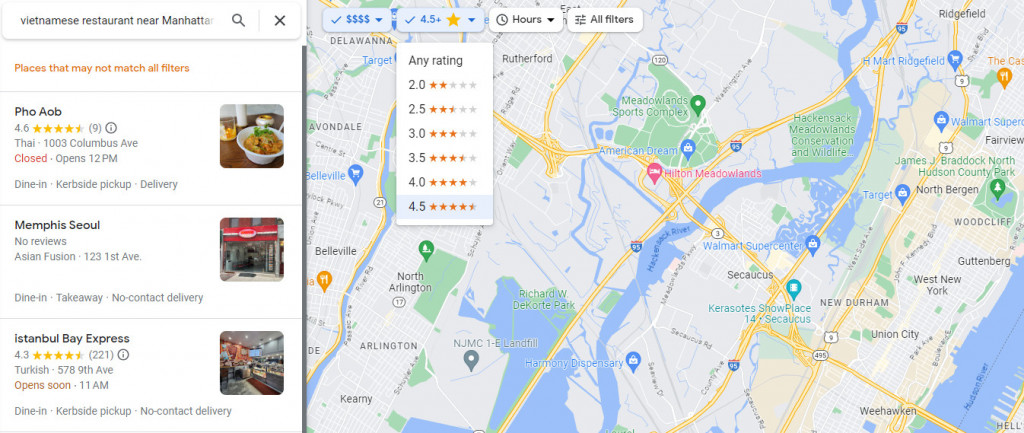A screen capture showcases a Google search for "Vietnamese restaurants near Manhattan." On the left side, there's a vertical list of various restaurants, and on the right, a typical Google Street View map displays the locations of these establishments in Manhattan. 

The top-left corner features a search bar with the query, and below it, a list of restaurants is displayed. The first restaurant listed is "POHAOB," a Thai restaurant located at 1003 Columbus Avenue, boasting a 4.5-star rating and currently closed, set to open at 12 p.m. The second listing is "Memphis Soul," an Asian fusion restaurant at 123 First Avenue, which does not have any reviews yet. The final restaurant in the list is "Istanbul Bay Express," a Turkish restaurant at 578 Ninth Avenue, with a 4.3-star rating, opening soon at 11 a.m.

To the right of the list, the Street View map of Manhattan shows the various restaurant locations, with an overlay featuring their ratings. The filter has been set to show restaurants with a minimum rating of 4.5 stars, which is highlighted in the drop-down menu, reflecting the user’s preference for highly-rated eateries.